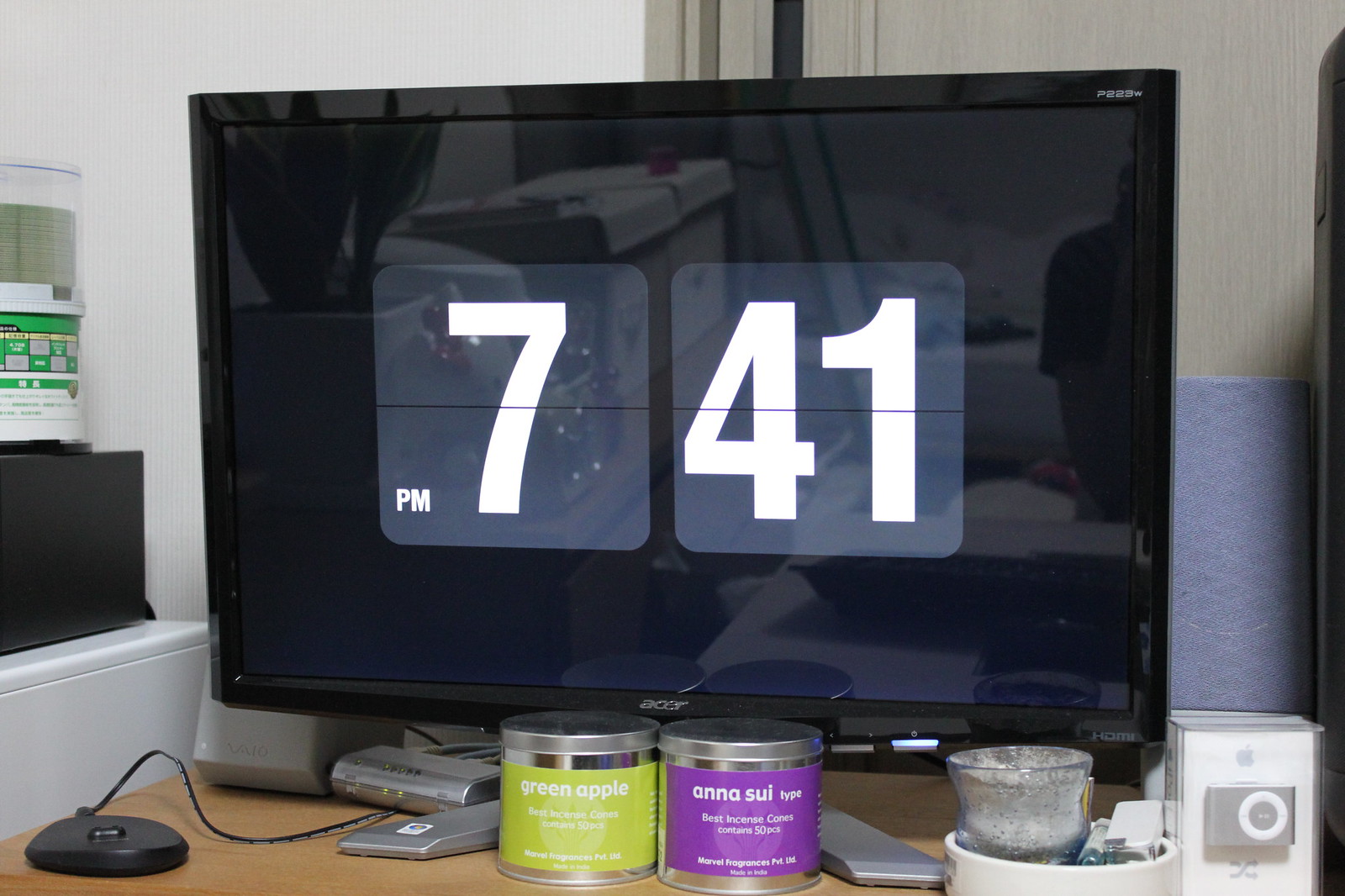The image depicts a detailed setup of a desk area with various objects and elements. Central to the scene is an Aspen monitor displaying the time as "7:41" on the left side. The monitor features two squares in the center, with the left square showing the number "7" and the right displaying "4.1". To the left of the monitor, a white wall and a gray door, possibly serving as a divider, are visible. 

On the left side of the desk, there is a tray containing a collection of CDs, along with a mouse possibly adjacent to it. A VAIO speaker is prominently positioned on this side as well. Two cans labeled "Best Incense Combs," containing 50 pieces, are placed in the front area of the desk. 

Adjacent to these cans, there is a green apple with a green label on the left and a purple (possibly another piece of fruit or object) on the right. To the far right of the desk is a container for incense and a lighter, next to which is a tiny Apple iPod Nano and another speaker. The monitor's screen displays a reflection of the room, adding depth to the image.